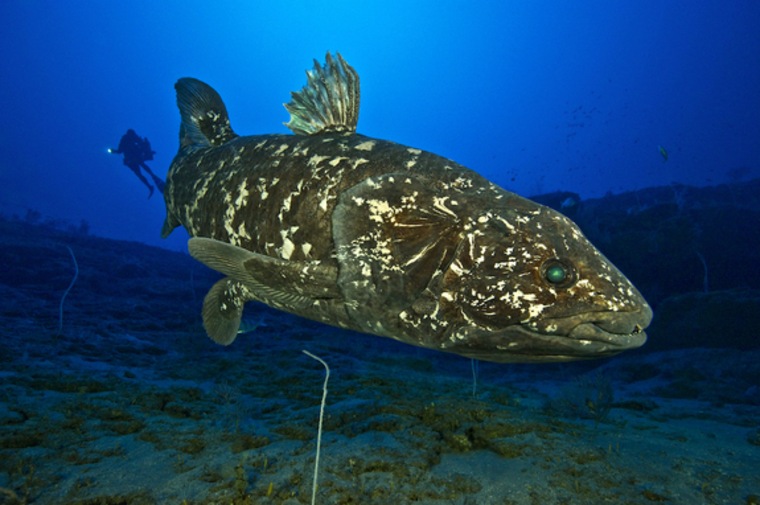This detailed underwater photograph captures a fish positioned centrally at the very bottom of the ocean. Illuminated by camera lighting, the fish is predominantly brown with distinctive mottled white markings and a striking green eye, possibly reflecting the surrounding water and seabed. From the side view, the fish’s body features a notable mohawk-like fin on its top and another fin near its anterior bottom. The ocean floor, visible not too far below, is scattered with rocks and patches of green algae, giving a blue hue due to the water's clarity. In the distant background, a scuba diver equipped with gear and large flippers is seen holding a light source but looking away from the camera. This diver, barely discernible in the image, adds context to the underwater scene, hinting at the presence of another diver taking the photograph.